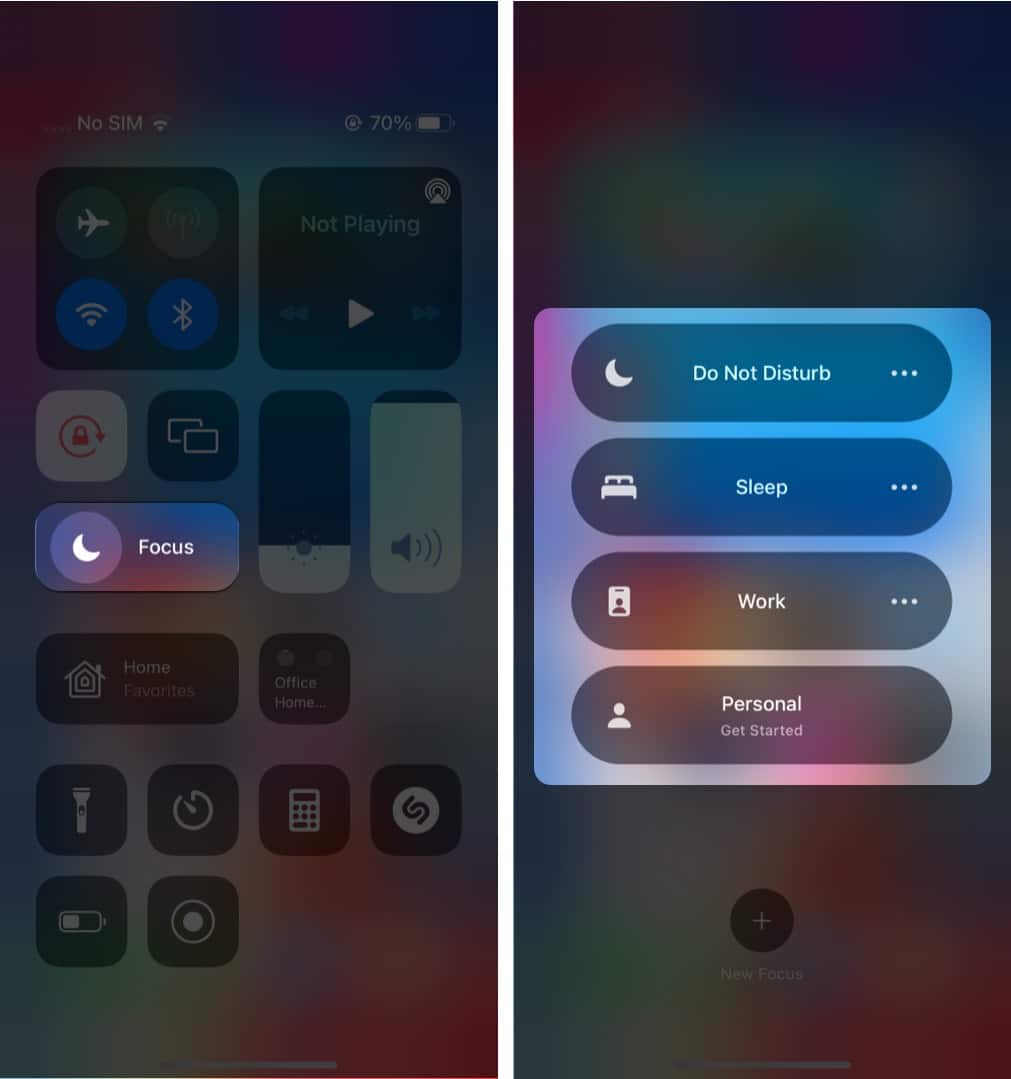This image captures the notification screen of an Apple device, showcasing its various functionalities. The screen displays a "No SIM" notification and shows a battery status of 70% along with being in Airplane Mode. There's a blurred option icon visible, as well as icons for Wi-Fi and Bluetooth all clustered in the same area, within a distinct square. 

Adjacent to this, in another square, is the music control interface. Though music is not currently playing, the interface includes arrows for previous and next track, replay, and a play button. Below the music control square, there is a volume control slider.

To the left of the volume controls are two icons for screen sharing and screen locking. Directly beneath these icons are the Focus mode options, represented by a moon icon, and a 'Home Favorites' icon. Adjacent to these, there is an 'Office Home' icon.

Also located on the screen are several utility icons arranged at the bottom, including the flashlight, clock, calculator, Shazam, battery indicator, and screen recorder.

To the right side of the image, the screen displays several focus functionalities including Do Not Disturb, Sleep, Work, and Personal options, with an option to 'Get Started'. At the very bottom, there is a plus sign labeled "New Focus" for adding new focus modes.